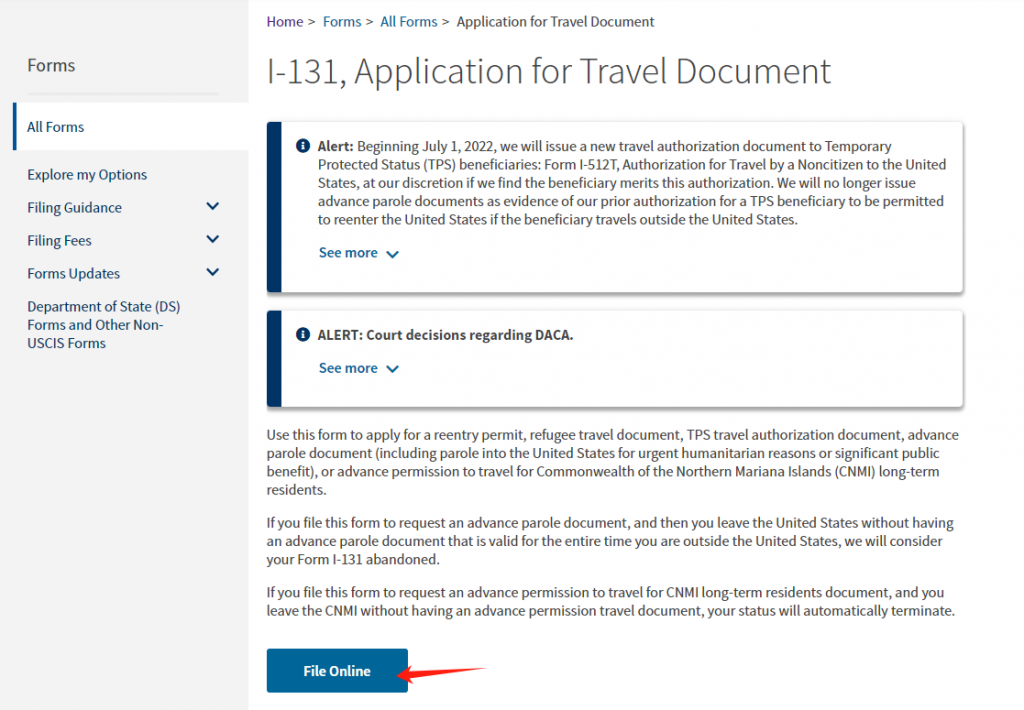Image Description: 

This image showcases a webpage featuring the I-131 Application for Travel Document form. The layout is clean and professional, predominantly utilizing a white background with black text, and accented with various colors for emphasis. 

On the left-hand side of the page, a vertical menu labeled "Forms" is prominently highlighted. Below this section, there are additional navigation options including "Explore My Options," a dropdown menu titled "Filing Guidance," "Filing Fees," "Forms Updates," and "Department of State DS Forms." 

Centrally located at the top of the page is the form header "I-131 Application for Travel Document." Directly beneath this header is an alert box marked by an exclamation icon. The alert informs users about a new travel authorization document that will be issued starting July 1, 2022, and provides a "See More" button for expanded details. Another alert box mentions a "Court Decision Regarding DACA," also with a "See More" option.

Below these alerts, a brief informative text explains that this form is used to apply for a re-entry permit related to refugee documentation. To assist users in navigating the page, a large blue "File Online" button with white text is prominently placed near the bottom with a red arrow to the right pointing towards it, drawing attention to this critical action button.

The overall design is structured for easy navigation and clarity, with the tab section on the left side marked in a lighter gray to distinguish it from the main content area.